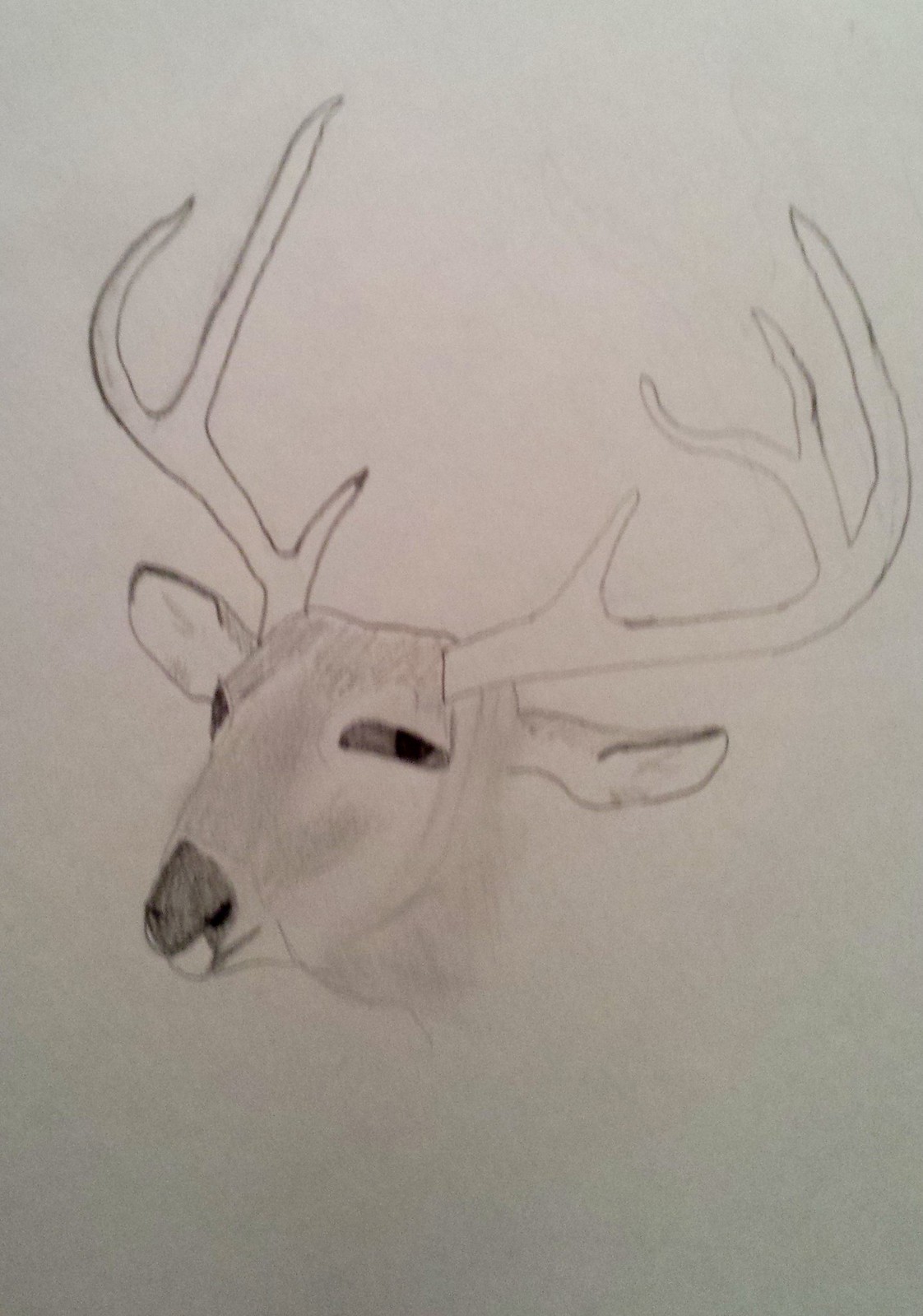This intricate pencil drawing on white paper features the head of a male deer angled to the left, yet appearing to gaze directly out at the viewer. The deer is centrally positioned on the page, with its neck fading out towards the bottom. The antlers are basic in outline, with the left antler having three points and the right antler exhibiting four points, extending symmetrically from the forehead towards the top left and right corners of the image. The ears, depicted with some shading, point straight out horizontally. The deer's face is detailed, particularly around the eyes and snout. The eyes are large and oval-shaped, with solid black pupils and grayish whites. The snout is dark, emphasizing the two black-shaded nostrils. The forehead is squared and angular, adding to the structured look of the jawline hints. The overall image is simple yet conveys a sense of depth through subtle shading and detail in key features such as the nose and eyes.